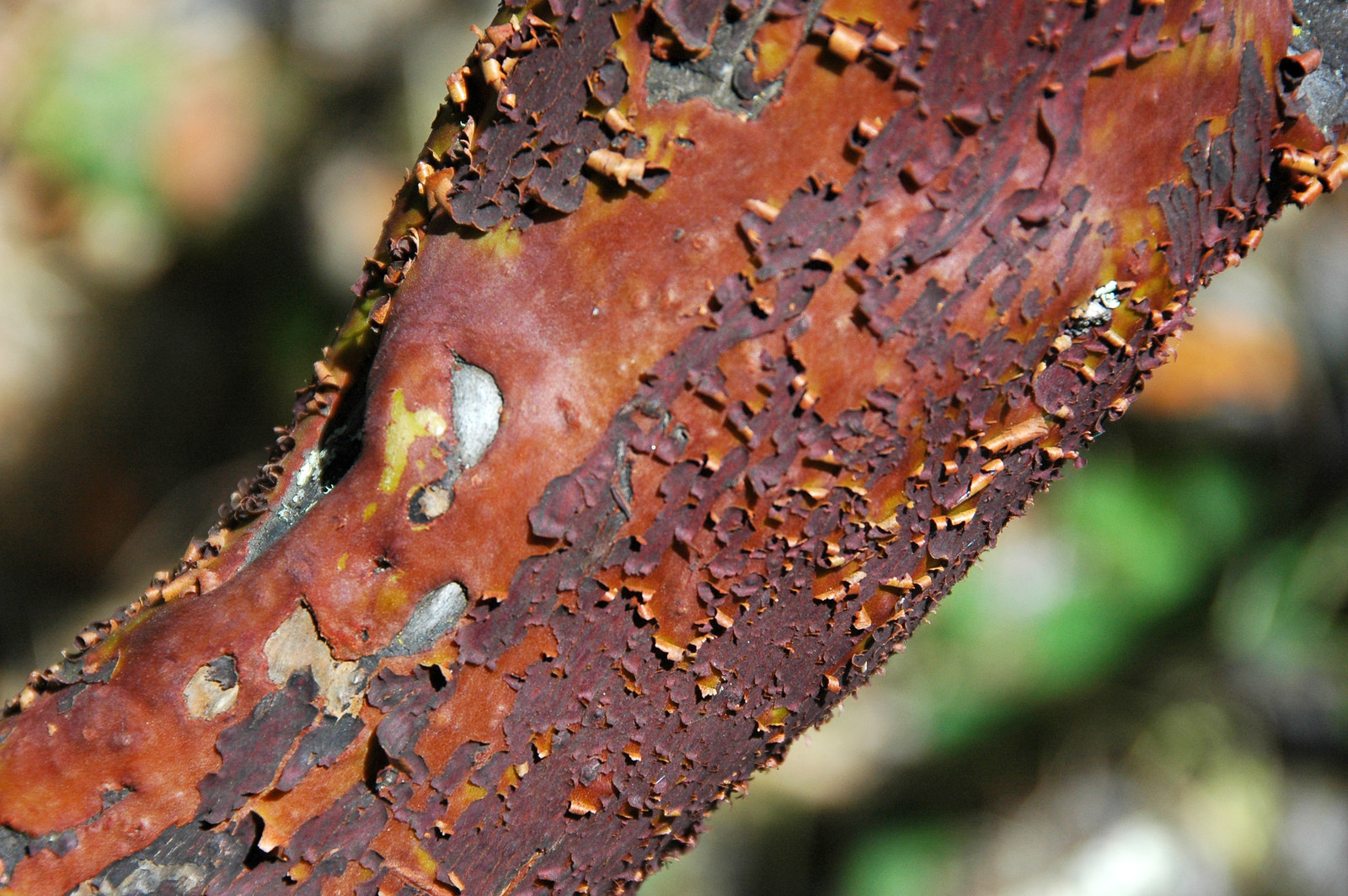This close-up image depicts a weathered tree branch with peeling maroon bark, revealing the orange-red wood and yellow undersurface beneath. Some sections of the branch show signs of damage, with nicks exposing a silvery layer of bare wood. The branch, which extends diagonally from the lower left to the upper right, features visible flakes and textures, suggesting the tree might be old or unhealthy. Behind the branch, blurred hues of green, orange, white, and black provide a colorful backdrop. The detailed zoom allows for a clear view of the intricate nooks and crannies, highlighting the textures and colors of the deteriorating bark.